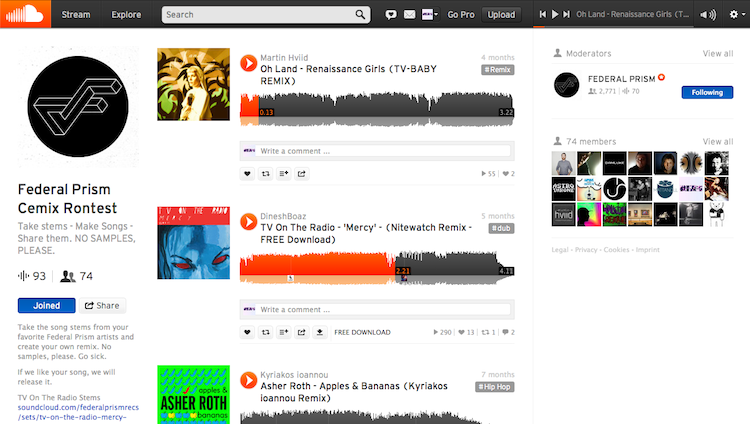In the upper left corner of the image, there is a smaller orange rectangle containing a white cloud with vertical white stripes on one half and solid white on the other. Below this cloud is a black rectangle with the word "stream" written inside. To the right of this, the word "explore" is displayed. Adjacent to this is an open white search bar, accompanied by options labeled "GoPro," "upload," and icons for rewind, play, and fast-forward.

Below this section, on the left, there is a black circle featuring 3D line elements resembling blocks. To the right of the black circle, there is an image of a woman’s face surrounded by some plants in the background, with the text "Martin HVLID" nearby. Below this text appears the song information: "Oh Land, Renaissance Girls, TV Baby Remix."

Directly below this, in a square frame, there is an image of a blue face with red eyes, followed by the artist title "TV on the Radio." The song title "Mercy" is placed in quotations, with "Nightwatch Remix" in parentheses and noted as a "free download."

At the bottom of the image, within a green square, the name "Asher Roth" is displayed. To the right, the text reads "Asher Roth - Apples and Bananas (Kyrakos LOANNOU Remix)," with a small gray rectangle underneath containing the hashtag "#hip-hop."